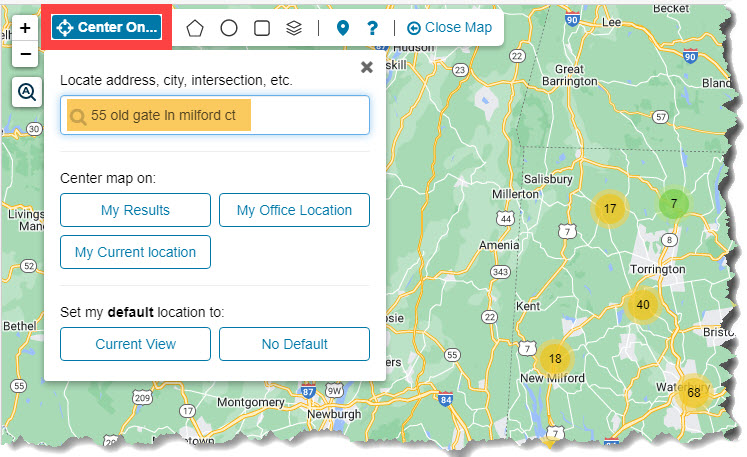The image displays a sophisticated site designed for locating specific addresses, cities, intersections, and more. Dominating the background is a detailed map featuring places such as Salisbury, Great Barrington, Beckett, and Torrington. Prominently displayed on the map is an example search for "55 Oldgate, Milford, CT," illustrating the site's capability to center the map on user-specified locations. 

Users can enter their desired location into a search dialog and adjust the map to center on the results, a specific location, or even their current location. The site also offers the convenience of setting a default location to be displayed each time the map is opened.

Along the top of the screen, a series of icons is present, including shapes such as a pentagon, circle, square, and a visually distinct icon resembling a small deck of cards. The exact functions of these icons are not immediately clear, as they lack accompanying text, but they are likely interactive tools that users can click to discover their purposes.

Additional features of the map include zooming capabilities, allowing users to zoom in and out for different levels of detail. There are also icons for obtaining help and for closing the map. The site's main logo is noticeably styled with white text embedded in a blue rectangle, accentuated by a thick red border, ensuring it stands out against the map's backdrop.